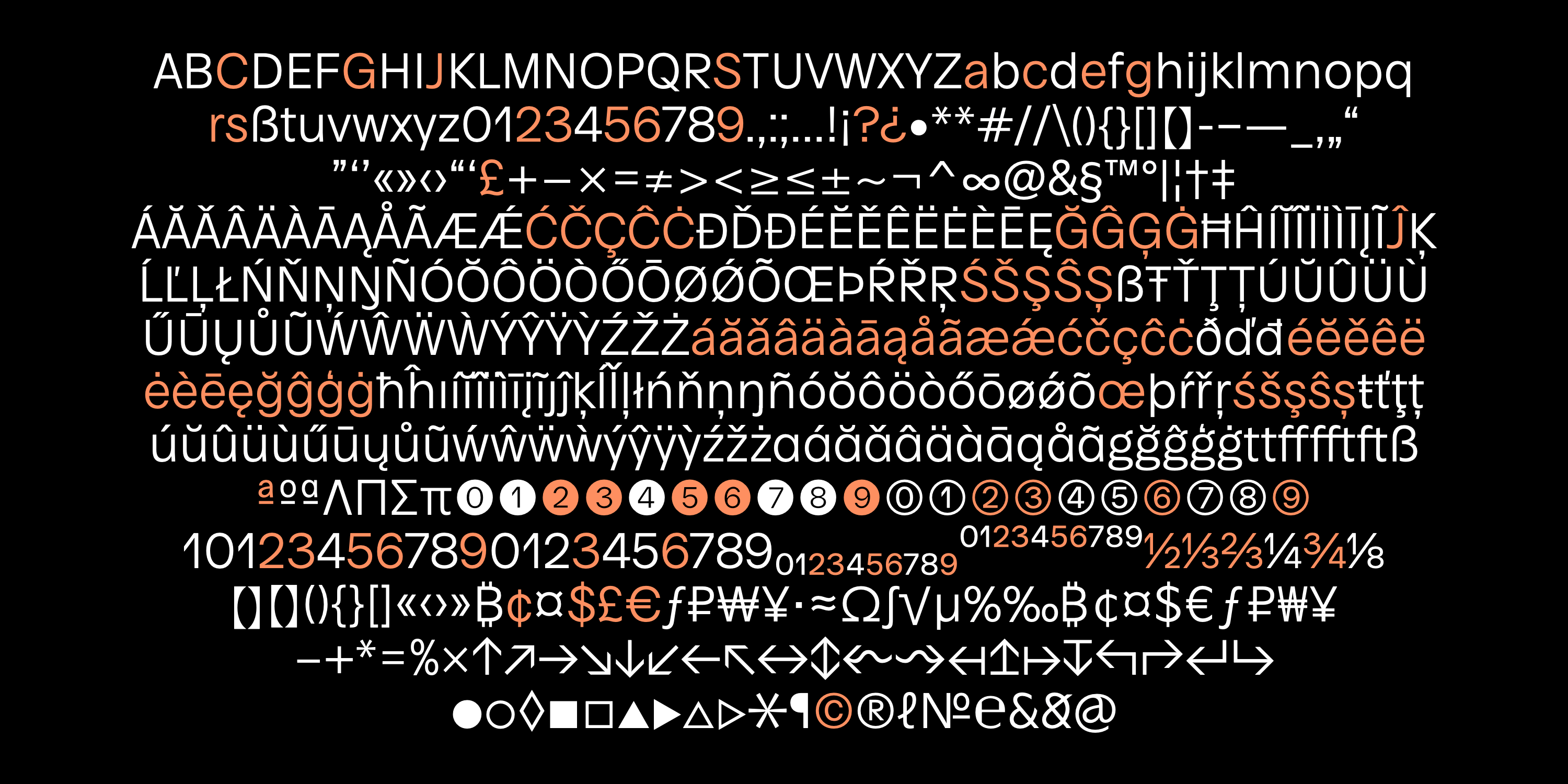The image features a black background adorned with a complex and organized array of letters, numbers, and symbols, spanning 13 distinct lines. The first line showcases the entire alphabet in capital letters, followed by lowercase letters starting from 'a' and ending at 'q'. Interspersed among these characters are sporadic highlights in orange, breaking the predominant white color without any discernible pattern.

The second line continues with 'r' and 's' and introduces a cursive 'b' before completing the alphabet with 't' through 'z', and includes digits from '0' to '9' along with a period and comma. Subsequent lines continue to vary, featuring a mix of standard symbols and accented letters, both uppercase and lowercase, over the next five lines.

Further down, the image displays a series of mathematical symbols such as the pi (π) and sum (Σ) symbols, alongside numbers encased in either filled or empty circles. It then transitions into fractions and various kinds of parentheses and brackets.

Additionally, the lower portion includes mathematical symbols like plus (+), minus (−), and asterisks (*), followed by an array of directional arrows pointing in multiple directions. The final row features fillable shapes such as diamonds, squares, and circles, completing the comprehensive collection of characters and symbols.